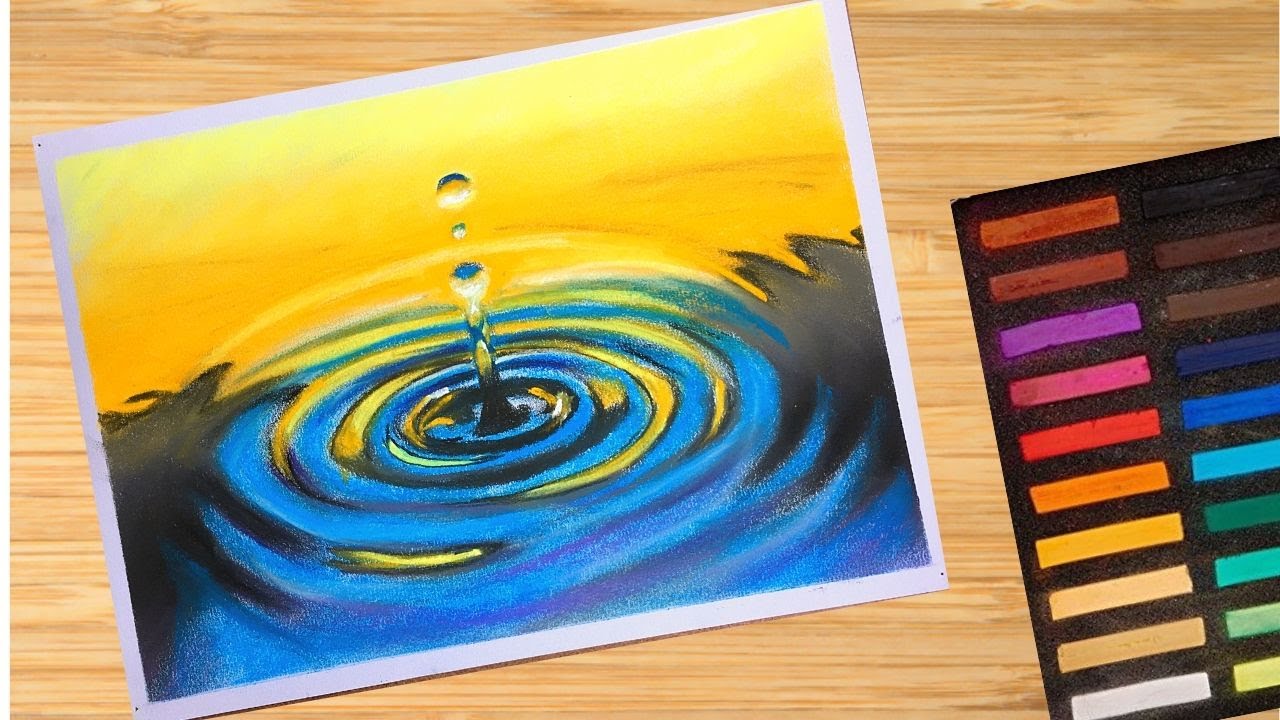The image depicts a rectangular landscape scene approximately twice and a half as wide as it is high, featuring a light wooden table with grain patterns stretching horizontally. On the left two-thirds of the image, a small rectangular illustration is prominently placed at an angle, tilting leftward about 20-30 degrees. This tilted illustration, bordered in white, portrays a drop of water splashing into a blue pool, causing a dramatic ripple effect. Concentric circles of blue and yellow radiate from the point of impact, crowned by a tower of water droplets extending upward. The background transitions from the blue water at the bottom to a yellowish sky at the top, hinting at a light source illuminating the scene.

Adjacent to this, on the right side of the image, a collection of multi-colored chalk pieces is aligned horizontally on a black background. This set, arranged at a similar leftward tilt, comprises two rows of pigments. The top row includes hues of brown, purple, pink, red, orange, yellow, and beige, while the bottom row features shades of black, brown, blue, teal, green, and yellow. These artistic tools, likely used to create the vibrant illustration, display an array of colors that mirror the diverse palette seen in the water and sky of the painting.